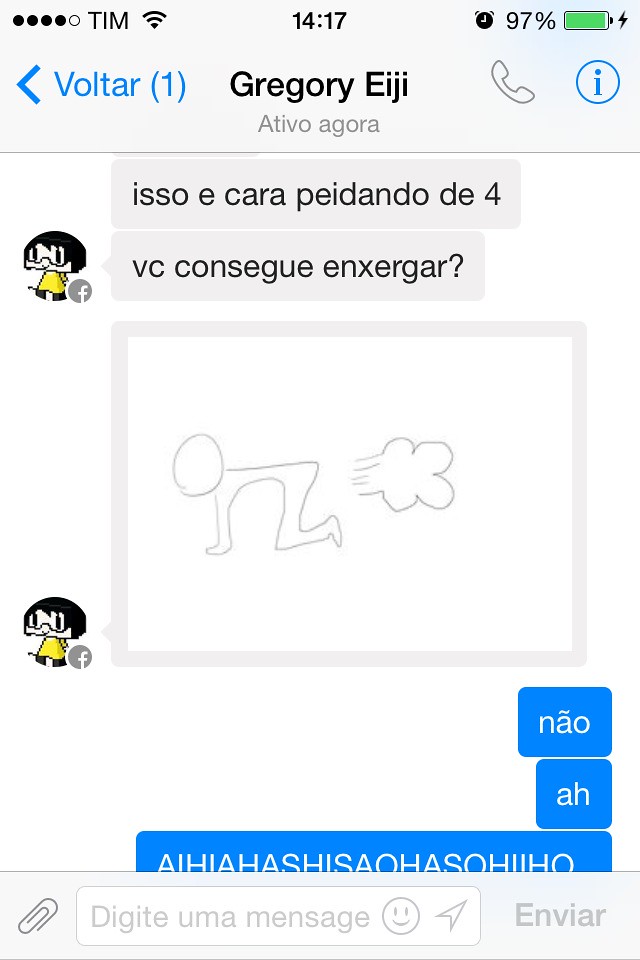The screenshot depicts a cell phone's interface with several distinct elements. At the top, the status bar shows the carrier "TIM," the time "14:17," signal strength represented by four black dots and one uncolored dot, and a battery icon at 97% power, colored green with a lightning symbol. Beside these, there's a small alarm clock symbol. Below the status bar, we see a blue left-pointing arrow next to the word "Voltar" in blue with a capital "V," and the number "1" in blue brackets. At the center, the name "Gregory Igey," spelled "G-R-E-G-O-R-Y-E-I-J-I," is displayed prominently with the text "Activo Agora" below it in a smaller font, suggesting his current activity status. 

The main content of the image appears to be from a text message conversation. The text in a gray speech bubble reads "Isso é cara peidando de 4? Vc consegue enxergar?" which seems to be in Portuguese, translating roughly to "Is that a guy farting on all fours? Can you see it?" This is accompanied by an illustration of a person bent over on all fours with a cloud behind them, indicating a fart. Below this, in a sequence of blue text bubbles, it reads "N-A-O" followed by "A-H," implying laughter or a response. Additionally, there's an emoji of a cartoon character with black hair and a yellow outfit beside the text bubbles, adding a humorous element to the conversation.